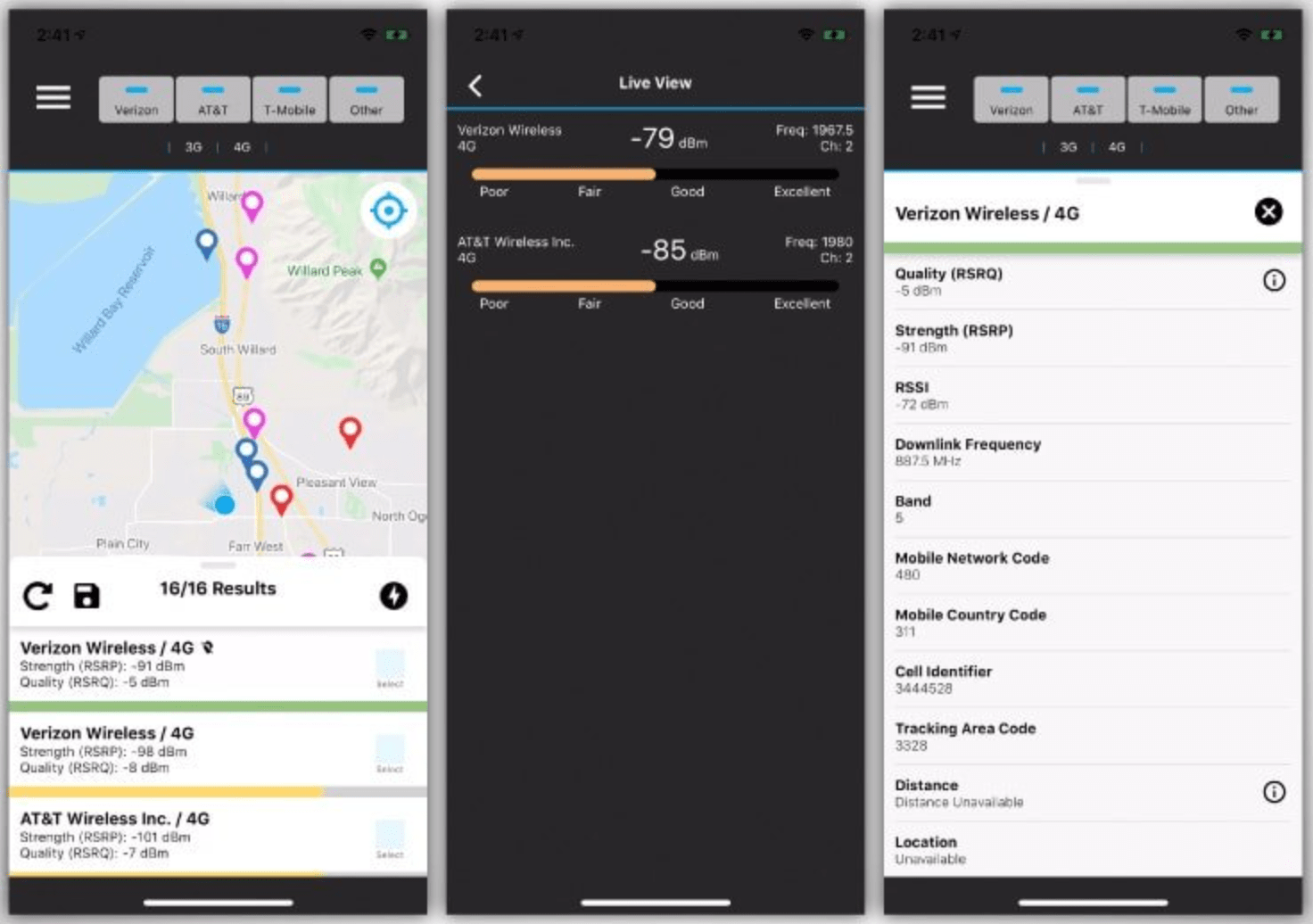This detailed image, approximately 30% wider than it is tall, is divided into three equal sections: left, center, and right, each separated by a gray bar and outlined in gray. 

**Left Section:** The left section features a digital map reminiscent of Google Maps, showcasing several pinned locations. There are three pins in pink, three in blue, and two in red. The map includes a body of water in the upper-left corner and a central north-south road flanked by most of the pins. The map displays "16 out of 16 results" as locations are listed vertically. These points appear to highlight areas with varying 4G signal strengths, noting Verizon Wireless 4G and AT&T Wireless Incorporated, along with detailed information on signal strength and quality.

**Center Section:** The center section is labeled "Live View," presenting two horizontal graphs. These graphs likely offer real-time data or visual representation of signal strength and quality across different locations.

**Right Section:** The right section is dedicated to detailed information on a specific signal site, marked as Verizon Wireless 4G. This section likely offers in-depth insights into the signal's strength and quality for that particular site, supporting the data provided on the map.